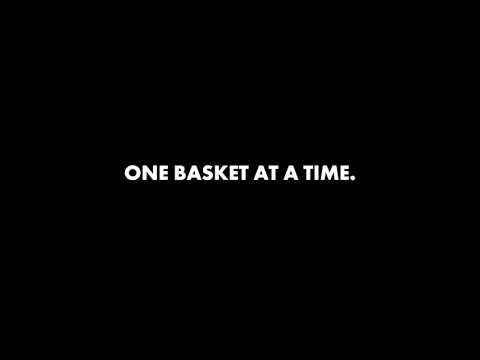The image is a minimalist graphic design with a solid black background in landscape orientation. Centrally placed in the frame, there is a single line of text in bold, white sans serif font. Capitalized and punctuated with a period, it reads: "ONE BASKET AT A TIME." The text, neither too large nor too small, is perfectly centered both horizontally and vertically, occupying about half the width of the image. The stark contrast between the black background and white lettering emphasizes the simplicity and impact of the design.